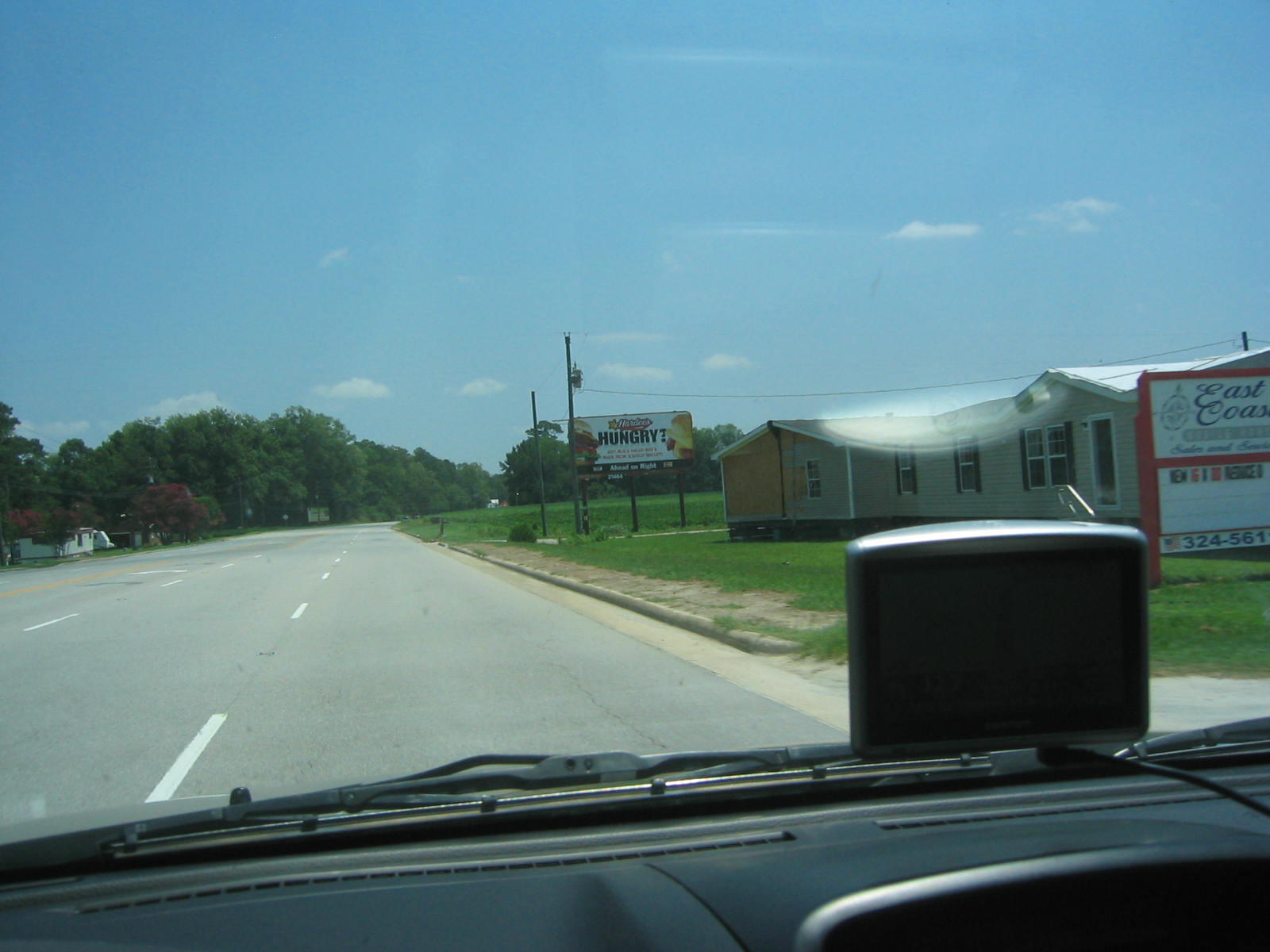In this image, a person is driving down a road in a car with a black dashboard, featuring a small device, possibly a GPS or a camera, mounted on top. To the right side of the road, there's a mobile home center with a notable sign: its border is red, the interior is white, and it contains blue letters with additional red text at the bottom. The mobile home center includes two light brown mobile homes, another large sign, several signposts, and a grassy area. The road stretches forward, lined with houses in the distance, under a clear, vibrant blue sky. The scene is framed by numerous trees, power lines, light poles, and a fence running parallel to the road.